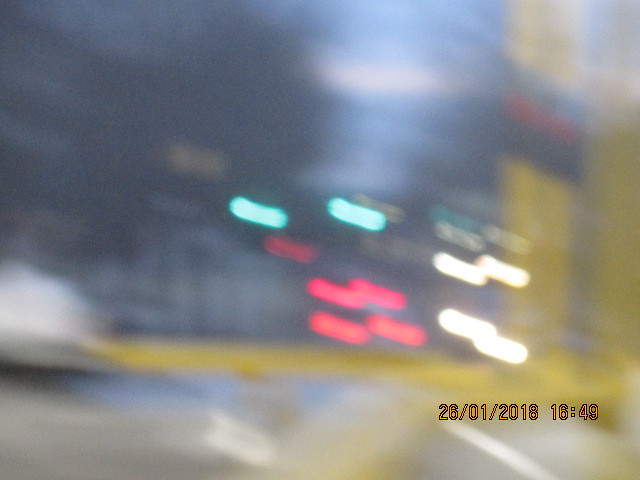A heavily blurred image, possibly depicting an outdoor or indoor scene, features streaking lights of red and white, likely from vehicle headlights and taillights, interspersed with light blue lights of uncertain origin. A thick yellow line, accentuated prominently on the ground, extends horizontally. This line is flanked by gray or darker surfaces. There appears to be a yellow pillar near the right edge of the image, distinguishable by a black stripe around its center, suggesting a caution marker for vehicles. To the left of this pillar, a large opening is visible, potentially serving as a passage for vehicles. The image bears a date stamp in orange text, reading "26/01/2018 16:49."